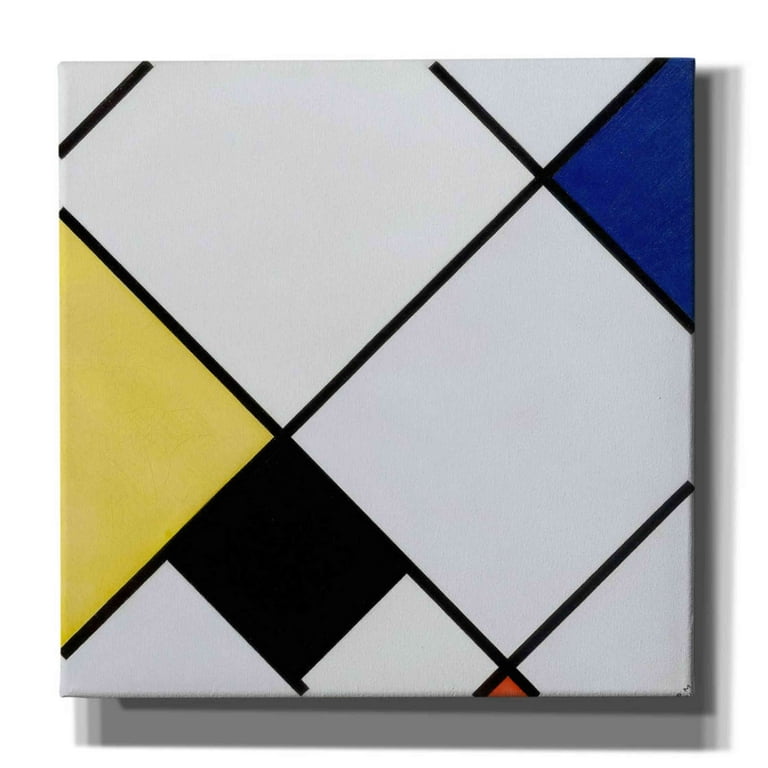The image features a photograph of a piece of abstract wall art designed to resemble a grid of tiles, each separated by black lines. Dominantly white, the composition includes partially visible colored tiles: a yellow one at the middle left, a blue tile in the upper right, and a hint of red starting to form at the bottom. Additionally, a small black tile is present. A thin gray border encircles the artwork, casting a shadow against the background. Despite the distinct primary colors and their cropped depiction, the black tile doesn’t conform to this primary color scheme, adding an intriguing element to the piece. The grid pattern and color placement evoke an abstract semblance to bathroom tiles.